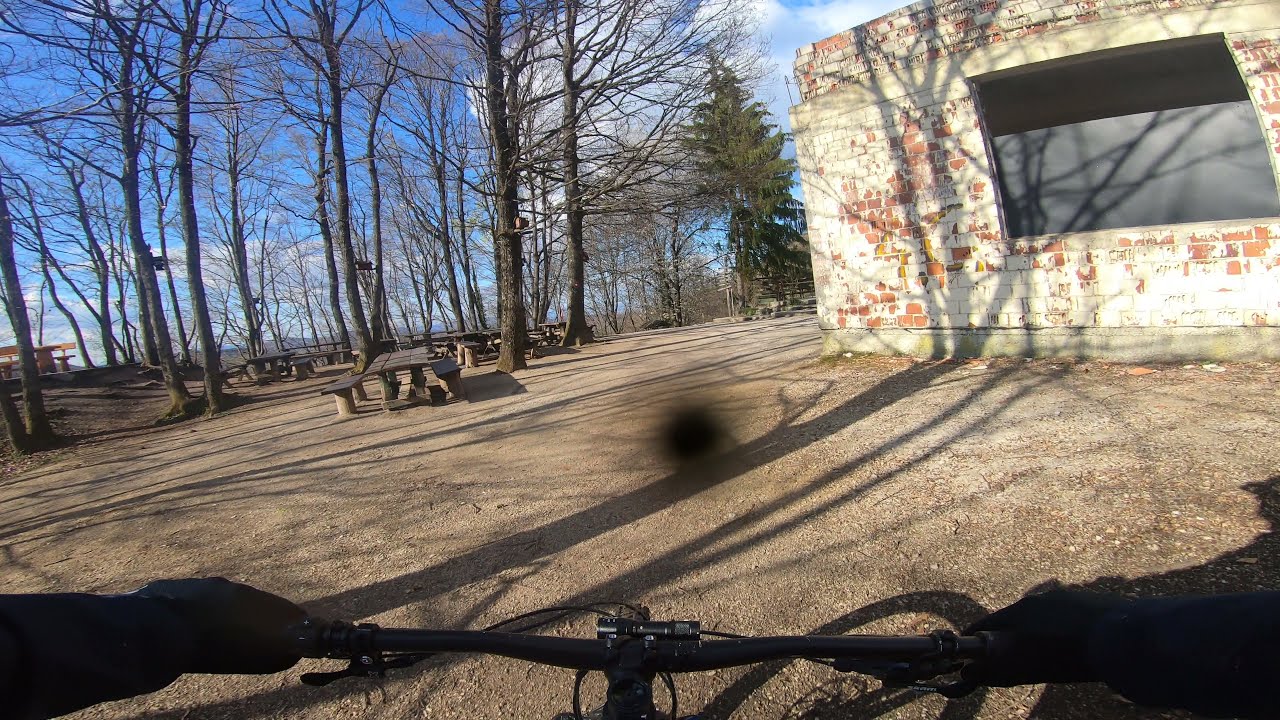Captured in a first-person view, this outdoor scene reveals a rider navigating a park on a mountain bike. The handlebars, brake levers, and the rider’s gloved hands gripping the black handlebars are prominently featured in the foreground. The rider appears to be wearing a long-sleeved dark shirt as they steer towards a picnic area. Scattered picnic tables rest under the leafless trees, conveying the wintry setting, with gravel covering the ground. The landscape features a mix of barren deciduous trees and a solitary pine tree, adding to the still, cold atmosphere. On the right side of the image stands an old, neglected concrete brick structure with what looks like an old concession window. Above, a blue sky with a few white, puffy clouds soars, casting a serene backdrop to the scene. The vivid earth tones—brick red, browns, greens, and blacks—along with shadows on the ground, complete the calm, deserted park ambiance.